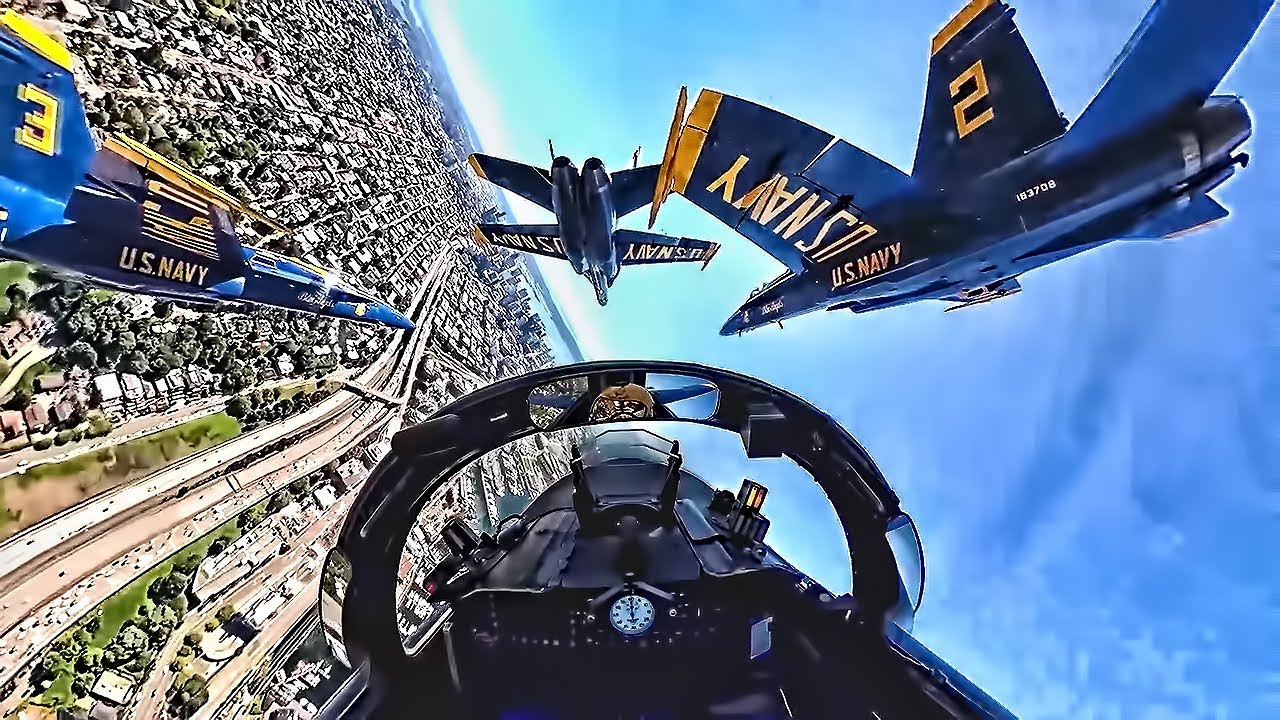This photograph, taken from the cockpit of a U.S. Navy Blue Angels fighter jet, captures the dramatic moment as the jet and its formation teammates perform synchronized barrel rolls. The viewer's perspective tilts diagonally, with the horizon almost vertical, as the jets bank hard to the left. Three other Blue Angels jets are visible, one ahead and two to the sides, flying in close formation. The jets are predominantly dark blue with striking yellow accents on the wingtips and bold yellow "U.S. Navy" markings on the sides and underneath the wings. Each jet is uniquely numbered on their vertical stabilizers, with numbers two and three discernible despite slight motion blur. Below, a sprawling cityscape with high-rise buildings and a winding highway is clearly visible, set against a distant waterway or ocean. The shot was taken through a cockpit window, evidenced by an arched connecting piece between the forward and rear glass panels, emphasizing the thrilling, immersive perspective of this aerobatic maneuver.